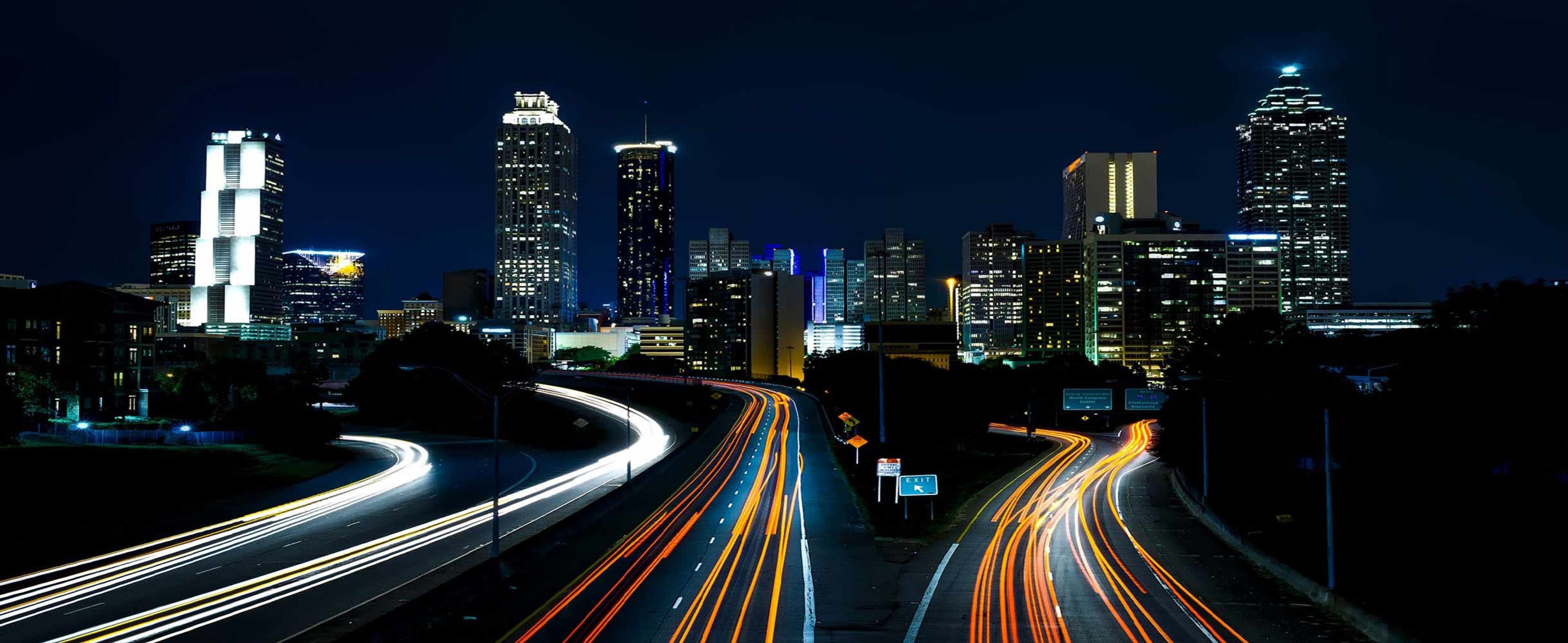This striking nighttime photograph captures a time-lapse of a busy downtown area featuring a multi-lane highway. The image reveals a total of six lanes, divided into three distinct sections, each glowing with the light trails left by speeding cars. The left section of the highway features two white light trails, while both the central and right sections display two orangey-yellow light trails each, all of which are the afterimages of car headlights, as no actual vehicles are visible.

Lining the highways, there are bright white and orange lights, adding to the dynamic feel of the scene. The center section also includes two orange construction signs, an exit sign, and an unreadable white sign due to the small text, while the right section has two street signs indicating exits.

The backdrop features a stunning skyline with approximately a dozen illuminated skyscrapers and various smaller buildings at their base, all set against a dark blue and black night sky, further emphasizing the vivid contrast of lights. There are no people visible, intensifying the focus on the bustling yet ghostly cityscape marked by the light streaks of countless cars zooming through the night.